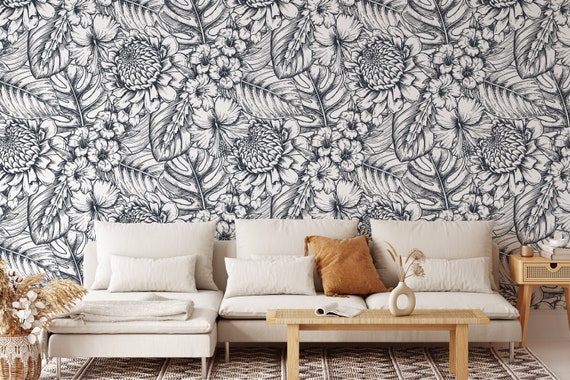The image captures a tastefully decorated living room where earth tones predominate. The central piece is a white arm-less couch adorned with seven pillows, one of which is brown. This couch is complemented by a small, light brown coffee table that supports an interesting flower arrangement in a unique bottle-like holder with a hole in the middle. Beneath the table lies a geometrically patterned rug in shades of brown and white. To the left of the couch is a beige potted plant, possibly artificial or dried, while to the right, a small beige side table stands. Dominating the scene, however, is the striking black and white wallpaper behind the furniture. This wallpaper features a detailed, repeating pattern of elaborately illustrated blooms and leaves, incorporating elements like small hibiscus flowers, large clover blossoms, daisy-like flowers, and ferns, giving the room a balanced yet eye-catching contrast to the earthy decor.